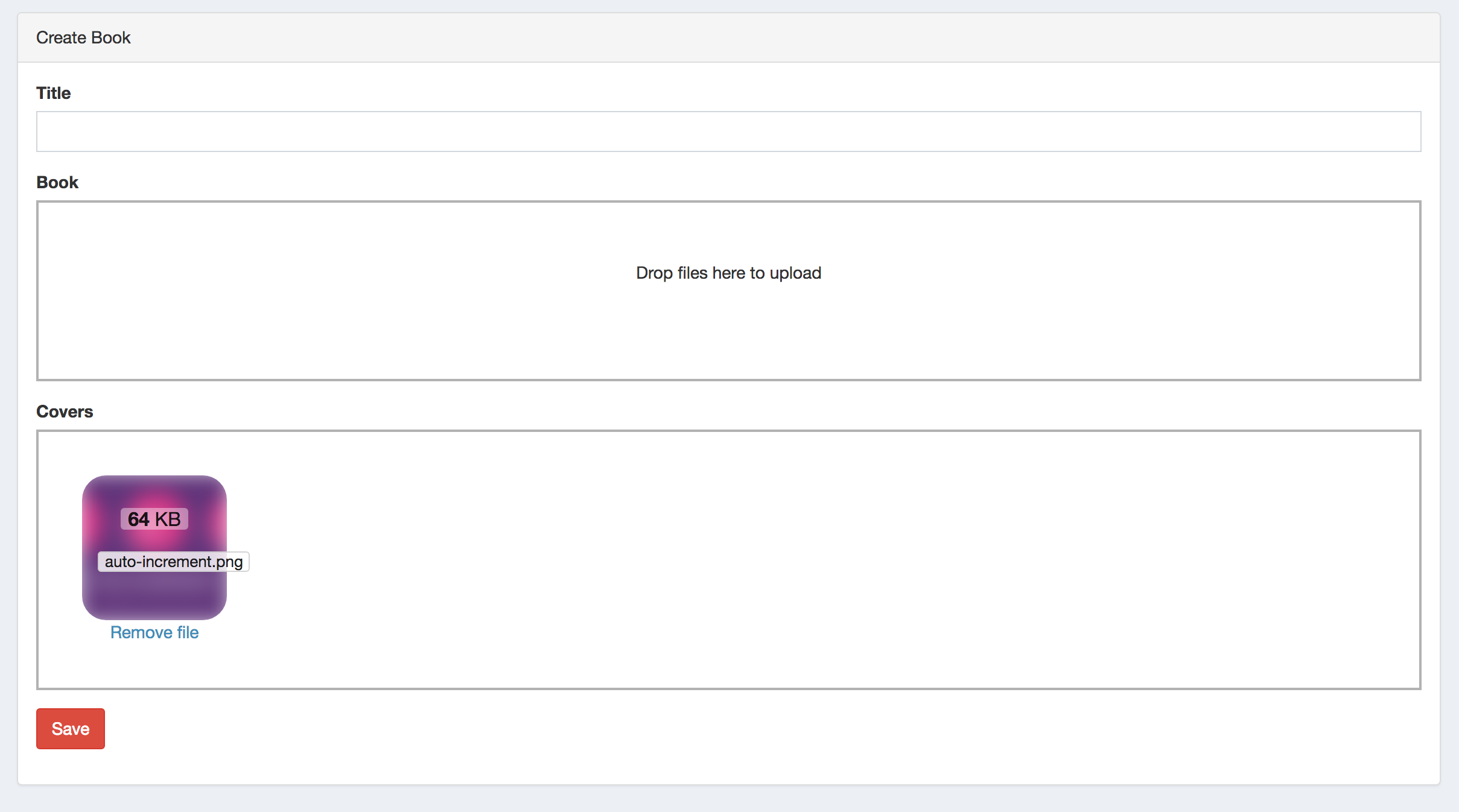In the image, we see a structured user interface designed for creating a book. The overall layout is enclosed by a large landscape area with a light gray border. The header section, slightly less blue-toned than the border, also adopts a light gray color. On the left side of the header, the words "create book" appear in a thin Arial font, rendered in black.

Proceeding downwards, the interface transitions into a white background. In the upper left corner, the word "title" is displayed in small black lettering. Adjacent to this is an elongated input field where users can enter the title of their book. This input field spans almost the entire width of the window and is encased in a light gray rectangular border.

Beneath the title input field, the text "book" appears towards the left in bold black lettering, again utilizing an Arial font. Below this descriptor lies a larger rectangular area surrounded by a medium gray border. This area contains the phrase "Drop files here to upload" in the same black font as the previous text.

Further down the interface, the word "covers" is displayed in bold black lettering using the same Arial font, positioned towards the left. This "covers" section is similarly surrounded by a medium gray border and maintains a rectangular shape. It is about 1.5 times larger than the area designated for book uploads.

To the left of the covers section, there is a prominently featured square icon with rounded edges, filled predominantly with dark purple. Towards the top of this icon, three fuzzy pink dots are visible, though the dots on the left and right are partially cut off, showing only about one-third of each. The central dot is fully visible. Overlaying this central dot is a transparent rectangular box with rounded edges, containing the bold black number "64." Adjacent to this number in non-bold black lettering are the uppercase letters "KB."